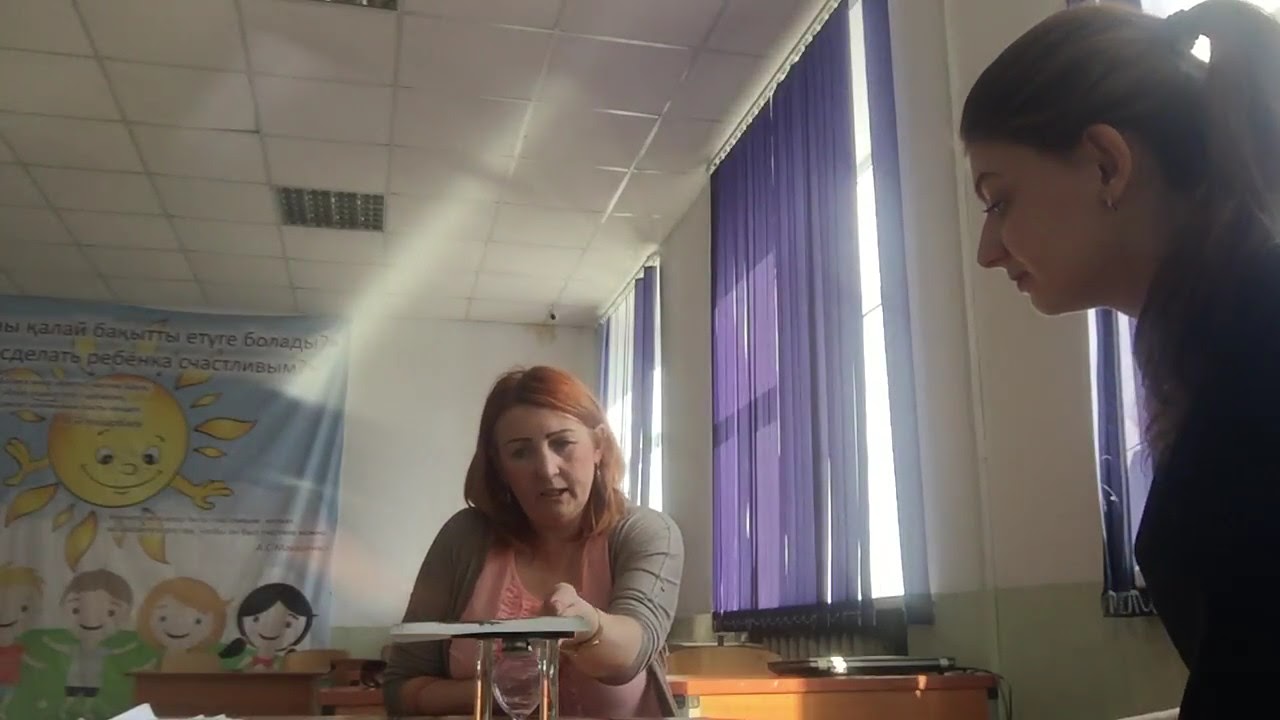The image depicts two women in a classroom setting with three windows covered by blue blinds that partially block sunlight, allowing just enough light into the room. Behind them are two wooden desks; one of them holds a laptop. The older woman, with red shoulder-length hair, is dressed in a pink shirt paired with a gray sweater, which is pulled up past her elbows. She appears to be placing a piece of paper over a glass object that resembles a stand with four glass tubes around the edges and a glass orb in the center. Nearby, a younger brunette woman with a pigtail is attentively watching the contraption. In the background, a large banner featuring animated images of four children standing in the grass under a sun decorates the wall. The boy on the left is partly cut off, while the other three children—two girls, one with red hair and the other with black hair, and a boy with brown hair—are fully visible. Some text in a different language is also present on the banner.